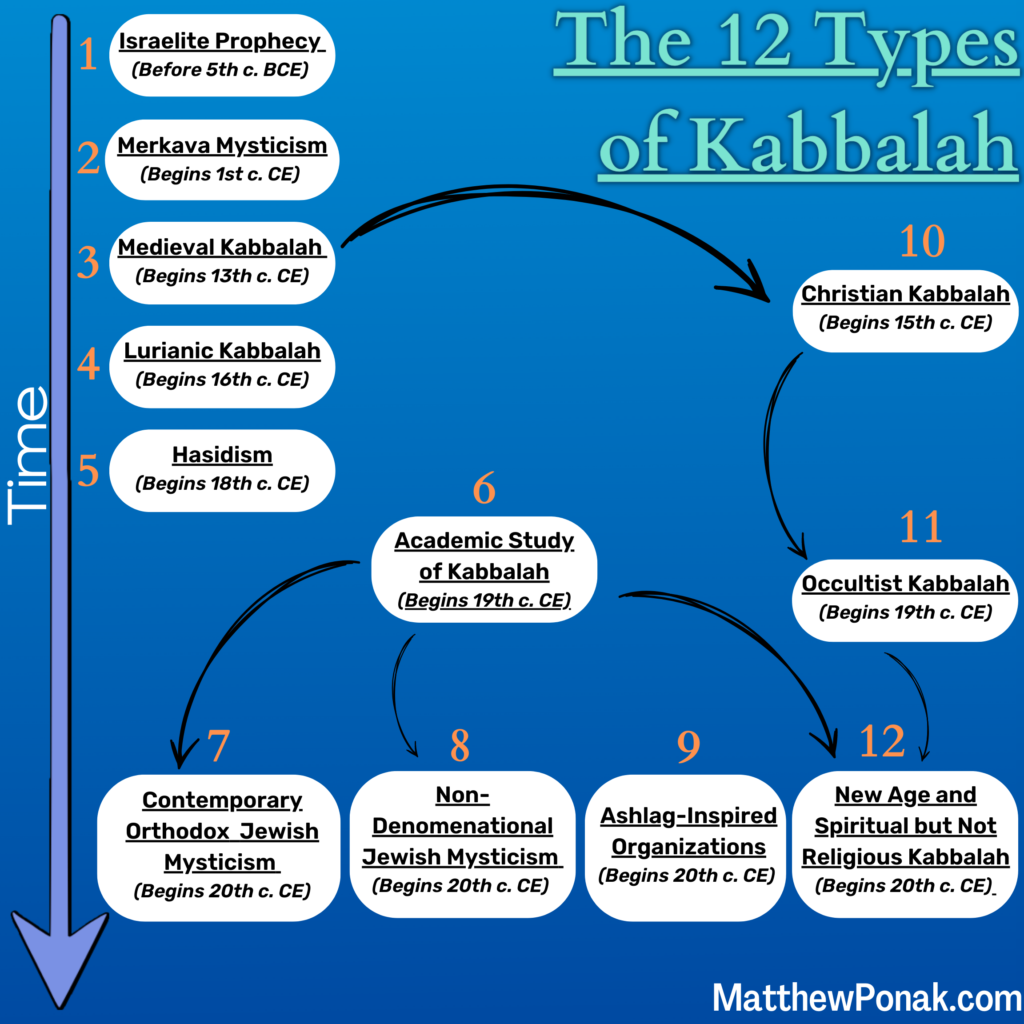The image is a detailed diagram of the "12 Types of Kabbalah" set against a gradient background transitioning from light blue at the top to a medium blue at the bottom. In the upper right corner, in teal underlined text, the title reads "The 12 Types of Kabbalah." A long purple arrow labeled "Time" runs vertically down the left side, indicating the timeline of the Kabbalistic traditions. The types are listed sequentially and positioned accordingly: 

1. Israelite Prophecy
2. Merkavah Mysticism
3. Medieval Kabbalah
4. Lurianic Kabbalah
5. Hasidism

In the middle, near the arrow, the 6th type is "Academic Study of Kabbalah." On the lower part of the diagram, aligned horizontally, are types 7 through 9: "Contemporary Orthodox Jewish Mystics," "Non-Denominational Jewish Mystics," and "New Age and Spiritual but Not Religious Kabbalah," with the 12th type at the farthest end. 

Types 10, 11, and 12 are positioned on the right side of the diagram. The individual types have been identified with corresponding sections: 

- "Christian Kabbalah" is near the bottom with number 10.
- "Occult Kabbalah" is listed as 11. 

Each Kabbalistic tradition is depicted in blues, blacks, light mint green, and light purplish blue colors. The diagram also includes various arrows, illustrating the chronological and categorical relationships between the different types of Kabbalah. Additionally, the bottom of the page features the text "MatthewPanik.com."